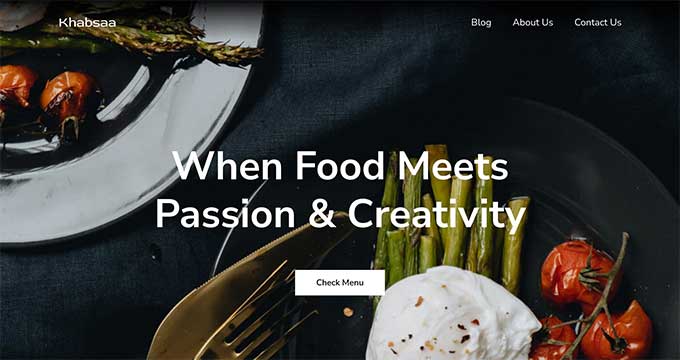The homepage of the Cabasa website (spelled K-H-A-B-S-A-A) prominently features the restaurant's name in white font in the top left-hand corner. Positioned on the top right-hand side, the navigation links for "Blog," "About Us," and "Contact Us" are also displayed in white font, albeit in a smaller size. Center-stage is a bold, white tagline proclaiming, "When Food Meets Passion and Creativity." Below this tagline, a white rectangular button with black text invites visitors to "Check Menu."

The background of the homepage showcases a visually appealing image of various dishes. Two plates are partially visible: the plate in the top left-hand corner is mostly cut off, while the other plate is more centered but still partially obscured. The top left-hand dish features roasted vine tomatoes and grilled asparagus, with a noticeable glare suggesting a white plate.

The second, more prominent dish is served on a blue plate, accompanied by a fork and a butter knife. This dish includes what looks like a fresh mozzarella cheese ball placed atop grilled asparagus, with vine tomatoes on the side. The image's appetizing layout and vibrant colors are designed to capture visitors' interest and whet their appetites.